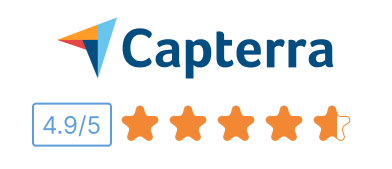The image showcases the branding and rating of a platform named Capterra. The word "Capterra," spelled C-A-P-T-E-R-R-A, is prominently displayed alongside a distinctive logo that resembles an origami arrow. This arrow is composed of multiple colored folds—specifically, orange, light blue, dark blue, and red.

Below the logo, there is a customer review rating system depicted using five stars, with the rating being an impressive 4.9 out of 5. Four out of the five stars are completely filled, while the fifth star is nearly filled, colored in orange. This rating is enclosed within a light blue outlined box. The image itself features a clean design with a white background, emphasizing the logo and the rating prominently. Despite lacking further contextual information, it suggests that Capterra could be associated with an app store or a review site due to its rating system.